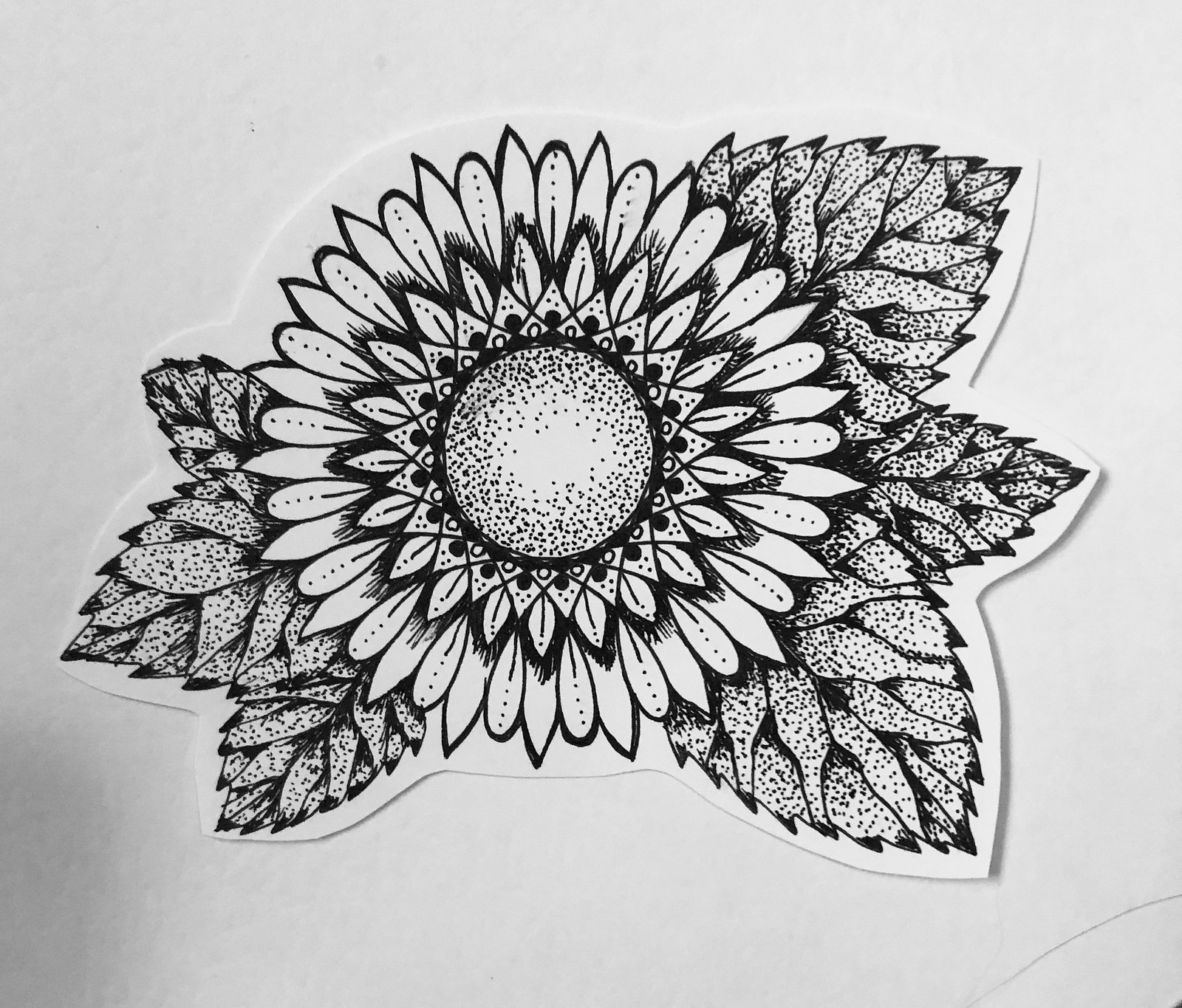In this image, we see an intricately designed black-and-white illustration that appears to be cut from a coloring book. The artwork, set against a stark white background, features a detailed depiction of a large flower with numerous small petals, meticulously rendered in black ink. Surrounding the central flower are several leaves, each filled with complex and textured patterns, further enhancing the visual richness of the composition. The precise lines and uniformity suggest that this piece was produced with print rather than hand-drawn, highlighting a professional and polished aesthetic. There is no text present in the image, allowing the viewer's attention to focus solely on the elaborate floral design and its decorative elements.